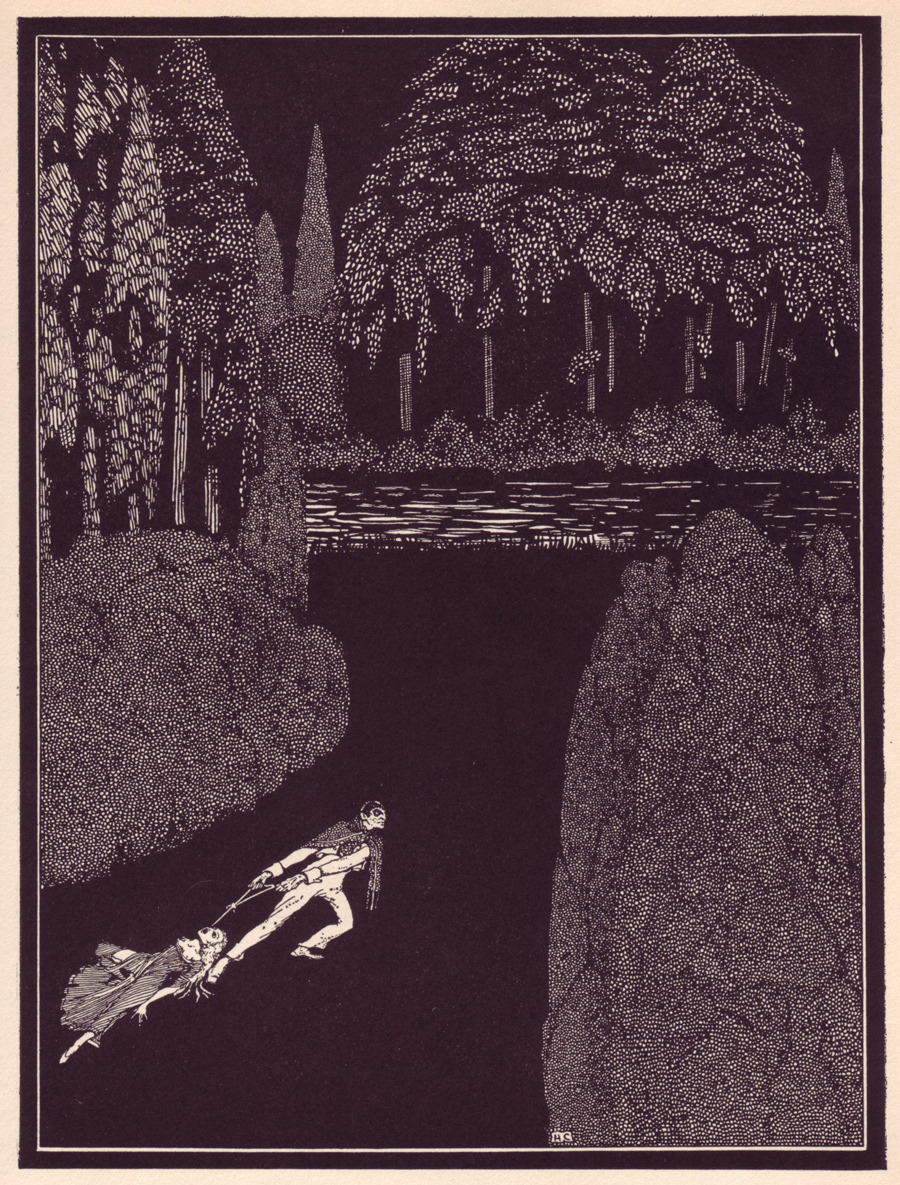This image, resembling a woodcut in its black and white execution, portrays a grim scene. Set against a dark, almost black background, the artwork features a stark contrast with white elements depicting an ominous forest with variously shaped trees surrounding the scene. A narrow path, set in dark tones, leads through the trees toward a white river that horizontally bisects the image. In the bottom left corner, a sinister-looking man, wearing a white suit and a black and white scarf or shawl around his shoulders, drags a woman by a rope tied around her neck. His face bears evil, horrific features, accentuated by his dark hair and nasty expression. He grips the rope with both hands, mid-step, moving towards the river. The woman he drags wears a black and white striped gown. Her body lies limp on the path, one leg splayed out and the other folded. Her long hair cascades along her left arm, which is outstretched on the ground, fingers clutching at the earth. Her eyes are wide open, mouth agape as if she is screaming or gasping. The entire scene is suffused with an eerie, gothic atmosphere, amplified by the monochromatic, high-contrast style of the woodcut.